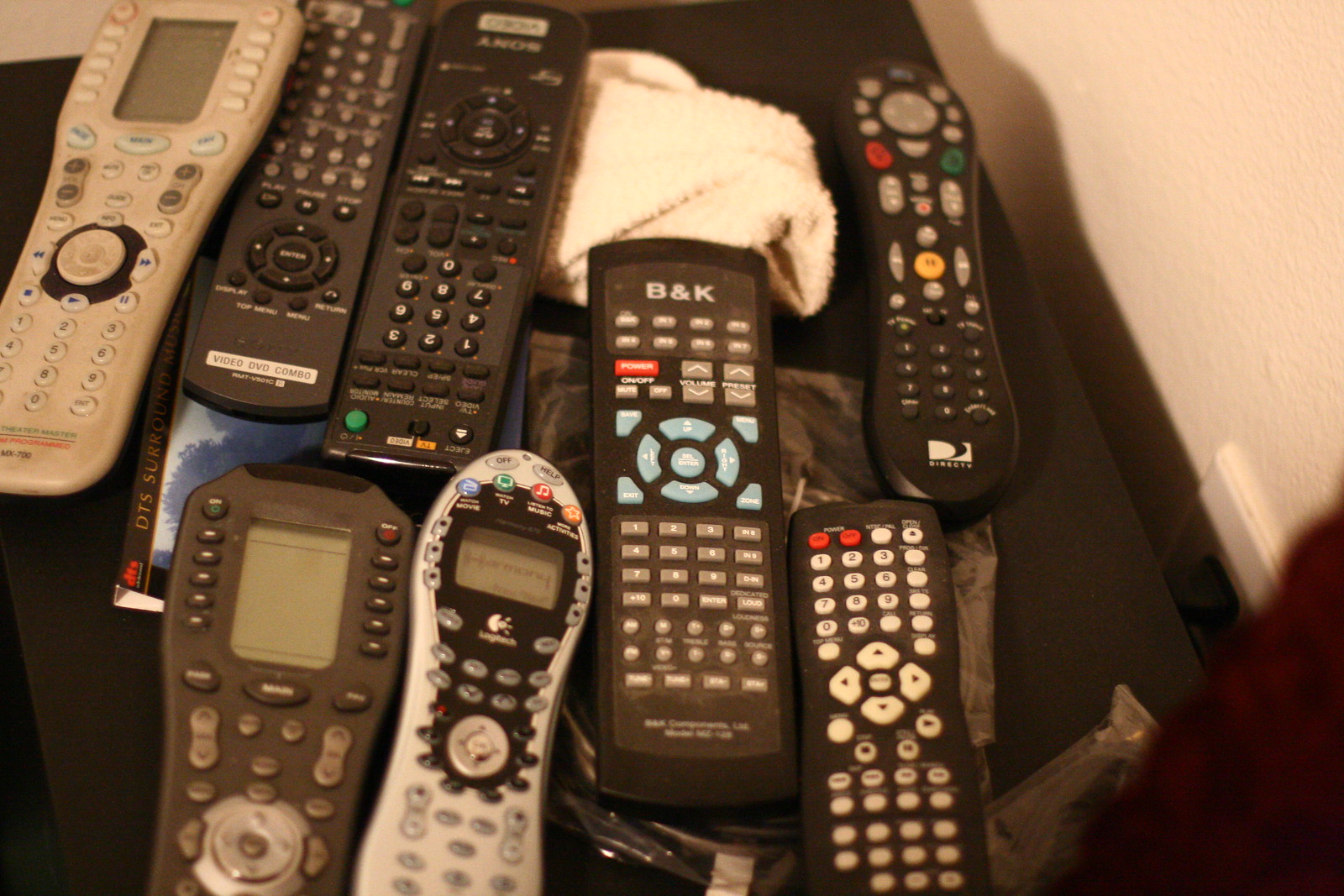The photograph depicts a collection of eight different TV remotes arranged on a black tabletop, most of which are black with a few exceptions. Notably, the remotes include a white one with a screen, a gray one with another screen, and variously shaped black ones. Among the remotes, brands like Logitech, Sony, B&K, and DirecTV are identifiable. Some remotes feature LED screens and keypads, with directional arrow buttons for navigation. The white washcloth and a magazine or label with a light blue pattern below the remotes add context to the otherwise technical setup. Additionally, in the right-hand side of the image, there's an outlet with a plug partially visible. Scattered among the remotes are objects like a book, a towel, and a cable wrapped in plastic.